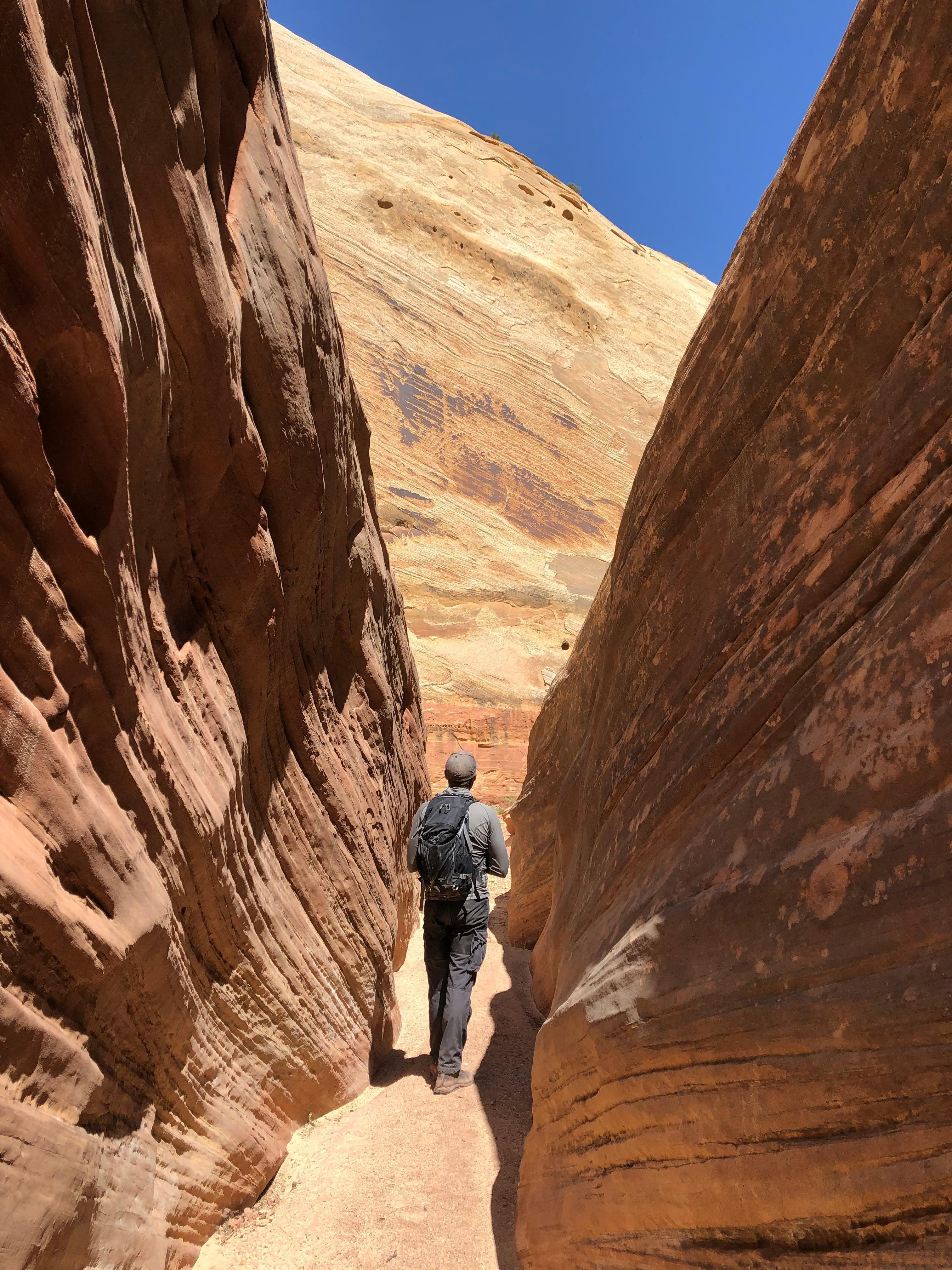In this captivating photograph, a solitary hiker, clad in a gray long-sleeve shirt, dark gray pants, and hiking boots, navigates a narrow passage flanked by towering rock formations. A small backpack, possibly a hydration pack, is strapped to his back, and a cap shields his head from the daylight. The trail is just wide enough for him to walk through and leads to another large, well-lit rock formation that contrasts beautifully with the clear blue sky above. The rugged walls, displaying striking strata and clay-colored hues with yellow tints, evoke the majestic scenery of the Grand Canyon or a painted desert. Though the environment lacks sandy expanses, its picturesque and awe-inspiring nature is undeniable, as the hiker ventures through this serene and breathtaking natural landscape.